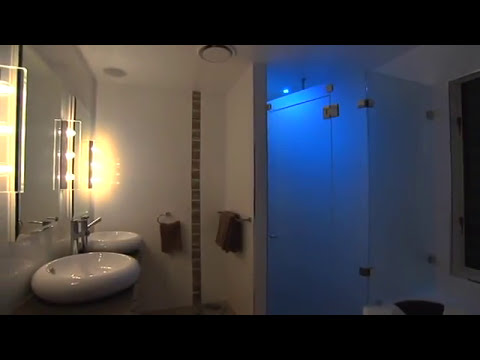This is a detailed photograph of a modern bathroom. On the left side of the image, there are two round, shiny white ceramic bowl sinks, each positioned below a large mirror. Flanking each mirror and positioned between them are vertical rows of three soft glowing yellow light bulbs, creating a warm ambiance. The walls behind the sinks feature a vertical backsplash that adds a touch of elegance. Adjacent to the sinks, you can see silver faucets and hand towel racks.

On the right side of the bathroom, there is a recessed area containing a clear glass shower door, behind which a bluish light from the ceiling creates a serene, glowing effect that contrasts the warm lights on the left. This area also contains towel hangers and a partially visible bathtub below the shower. The overall walls of the bathroom are white, adding to the clean and modern aesthetic. Additionally, a medicine cabinet with a mirrored door can be seen on the right, further enhancing the functionality and sleek design of the space.